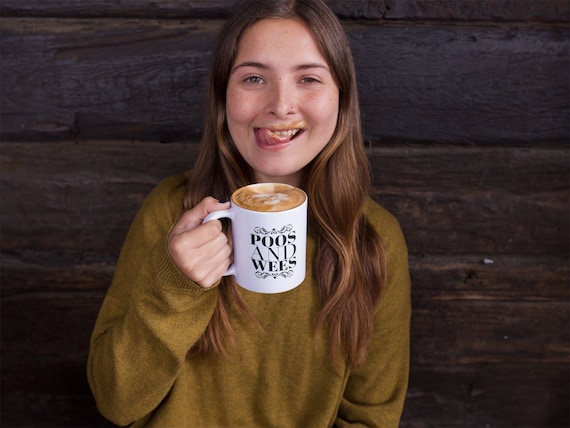The image is a clear and brightly lit horizontal landscape, depicting a young girl approximately 10-12 years old with long brunette hair and neatly groomed eyebrows. She is sitting in front of a dark brown wooden wall, which consists of boards stacked one on top of another, providing a rustic backdrop. The girl is wearing a long-sleeve mustard-colored sweater and appears happy as she looks towards the camera, with a hint of a smile and her tongue over her teeth, possibly licking away foam from her beverage. She holds a white mug with her right hand, which features black calligraphy that reads "poos and wheeze." Inside the mug is a drink with latte art, suggesting a hot chocolate or coffee. The image is very clear, with no other individuals or objects present, focusing solely on the girl and her moment of joy.